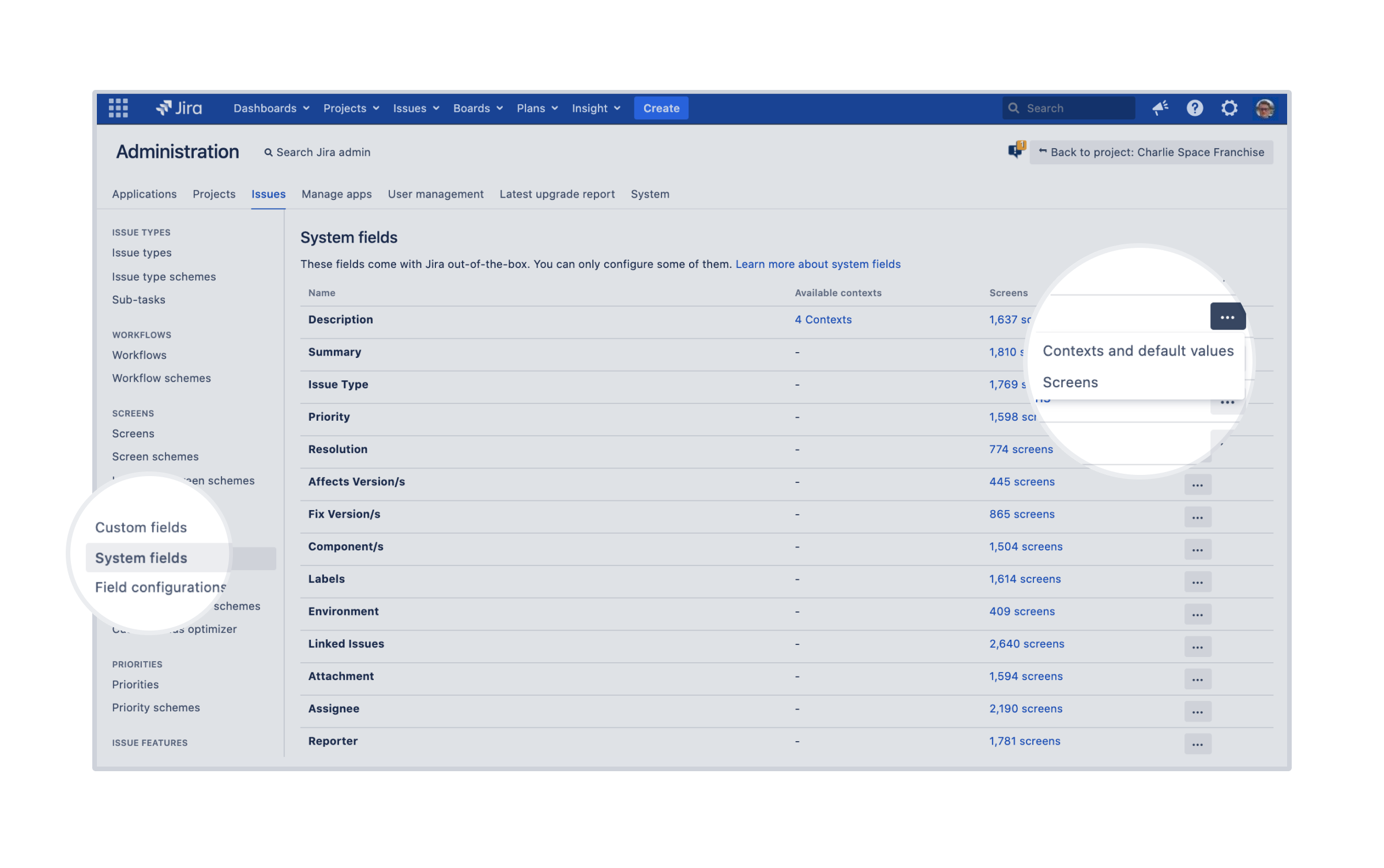The screenshot features a detailed view of a JIRA interface. At the top of the page, a blue banner spans horizontally, containing several key elements. 

In the upper left-hand corner, there is a square icon with three rows of three blocks, colored in light blue or gray. Adjacent to this icon, to the right, is a logo made up of three triangular shapes pointing diagonally to the upper right, accompanied by the text "JIRA." 

The main navigation menu is laid out horizontally along the blue banner and includes the following options, each with drop-down menus: Dashboards, Projects, Issues, Boards, Plans, Insight, and Create, with the "Create" option outlined in blue for emphasis.

On the upper right side, the interface displays a search bar. Following this are several icons: a speaker or bullhorn, a question mark, a widget, and finally a round profile picture of a male with short dark hair.

Immediately below the blue banner, starting from the upper left corner, the text "Text" appears, with another search bar labeled "Search JIRA Admin" positioned to the right. 

On the right side of the page, there is a black speech bubble icon with an exclamation mark in the center, next to a rectangular box that states "Back to Project Charlie Space Franchise."

Directly underneath is another horizontal menu with options: Applications, Projects, Issues, Manage Apps, User Management, Latest Upgrade Report, and System. 

On the left side of the screen, vertical options are listed, expanding from the top down: Issue Types, Issue Type Schemes, Subtasks, Workflows, Workflow Schemes, Screens, Screen Schemes, Priorities, Priority Schemes, and Issue Features.

A central round overlay on the left side highlights text options: Custom Fields, System Fields, and Field Configurations. The line for "System Fields" has a distinctive gray background.